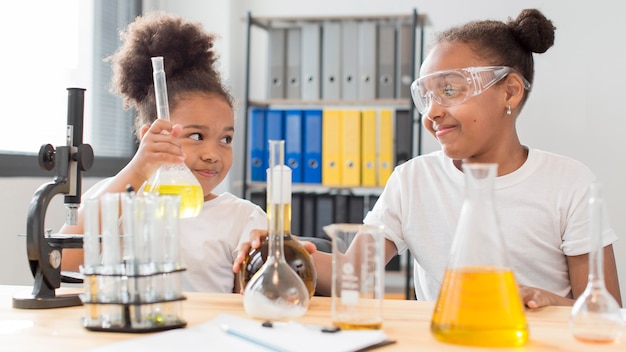In this detailed image, two young black girls are seated at a wooden desk in a science lab, deeply engrossed in a science project. Both girls are smiling and looking at each other, conveying a sense of enthusiasm and camaraderie. The girl on the left is slightly younger and is holding a beaker containing a yellow substance, while the girl on the right, who has her hair up in a bun and is wearing safety goggles and earrings, has her hand on another beaker filled with a brown liquid. The desk is cluttered with various scientific instruments, including multiple beakers with yellow liquids, a microscope, and possibly a telescope on the left side. Scattered around them are tools like round-bottomed flasks, a folder, paper, and pencil, creating a typical bustling lab environment. In the background, a shelf holds various colored binders in gray, blue, yellow, and black, and a window can be seen on the left, adding depth to the space. The two girls, dressed in white shirts, are clearly engaged in their experiment, capturing a moment of joyful learning and scientific inquiry.